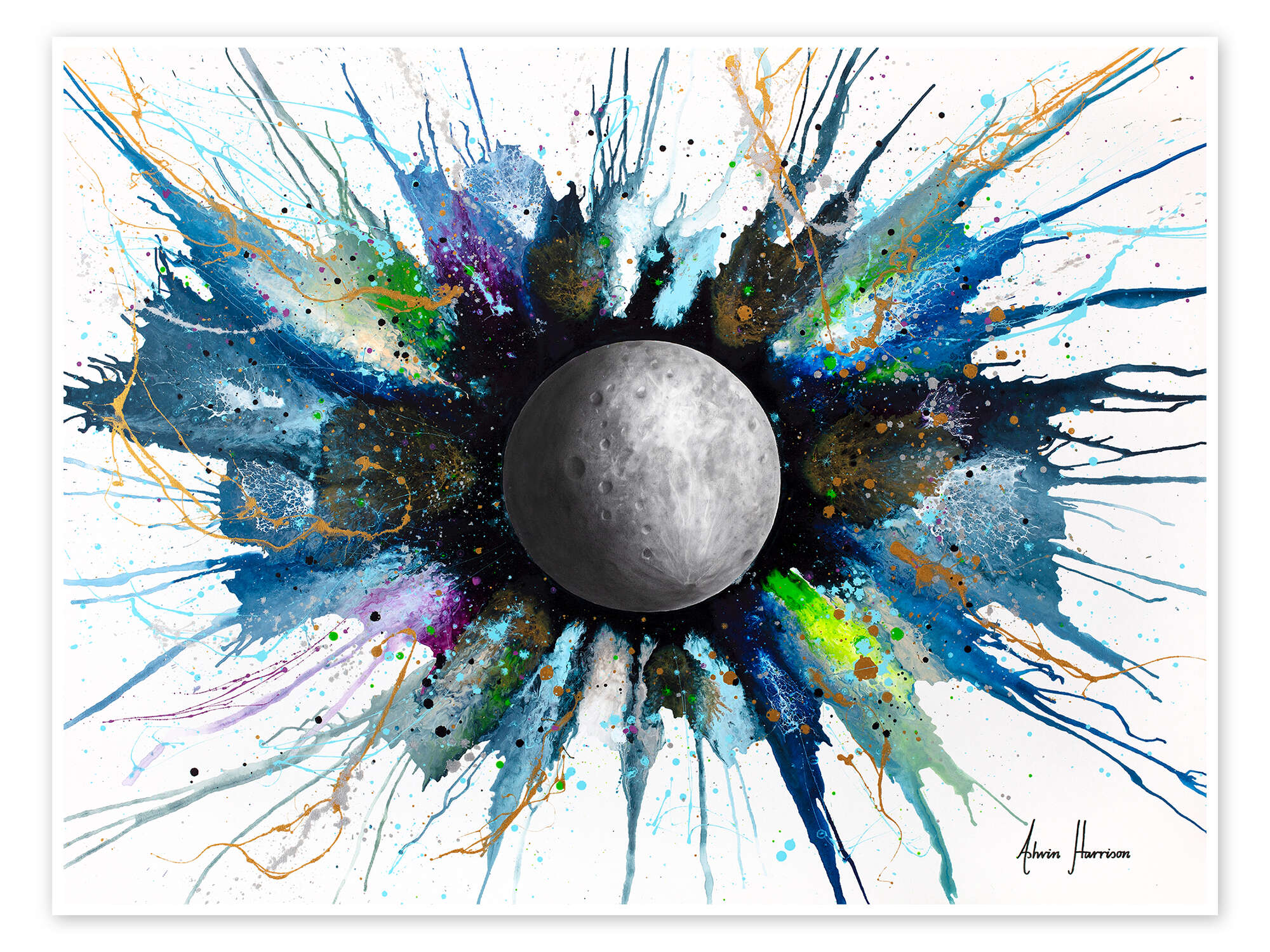The image features an abstract painting on a white background that prominently showcases a central, mottled gray circular form resembling the moon or a gray planet. The moon is detailed with various shades of gray, depicting its characteristic holes and indentations. Surrounding the moon, a dense black outline enhances its 3D effect, creating the illusion of depth. Radiating from this central moon figure, splattered paint in a myriad of colors—blue, green, purple, gray, light brown, gold, yellow, orange, and black—stretches outward in all directions, gradually thinning towards the edges. Notable highlights include brighter blue splatters at the upper right, lime green at the lower right, and some purple on the left. The black background interspersed with colorful splatters suggests the starry expanse of space. The painting is signed in black script at the lower right by the artist, Harrison.